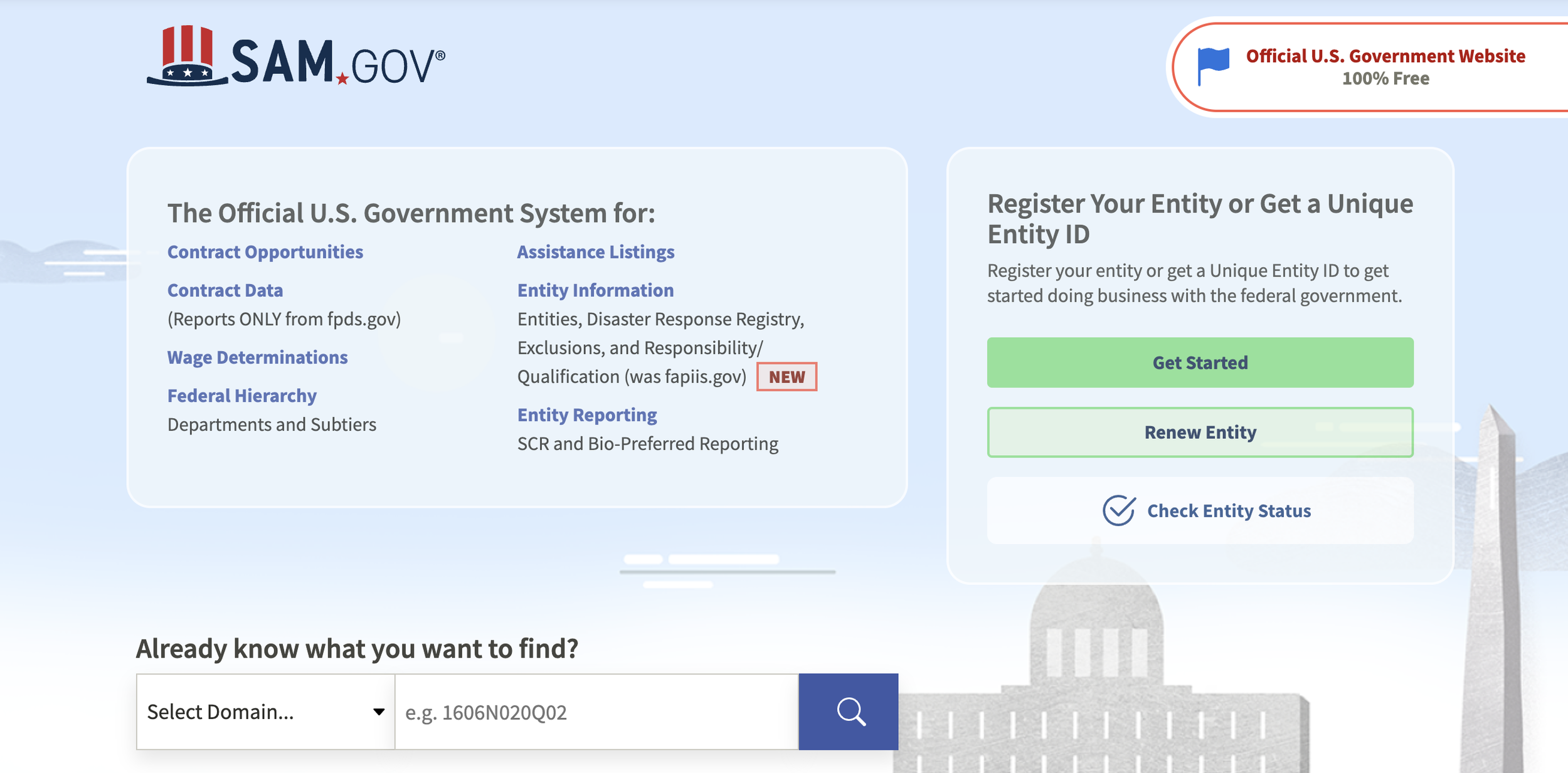This screenshot is from Sam.gov, an official U.S. government website that is entirely free to use. 

In the upper portion of the image, the Sam.gov logo features an Uncle Sam-style hat, characterized by its blue base adorned with white stars and vertical red and white stripes extending upward, reminiscent of both Uncle Sam and Abraham Lincoln's iconic headwear.

The text beside the logo articulates the website's purposes and services: "The official U.S. government system for contract opportunities, contract data, reports (only from FDPS.gov), wage determinations, federal hierarchy, departments and sub-tiers, assistance listings, entity information, entities, disaster response registry, exclusions, and responsibility/qualification." Below this enumeration, a note stating "That's new" is prominently displayed.

Underneath, the page instructs users to select a domain from a drop-down menu, offering an example number for guidance, along with a search icon. Further instructions advise users to "Register your entity or get a unique entity ID to start doing business with the federal government," followed by options to "Get started," "Renew entity," or "Check entity status."

At the bottom of the screenshot, there are cartoon depictions of notable Washington, D.C. monuments, adding a visually engaging element to the website’s interface.